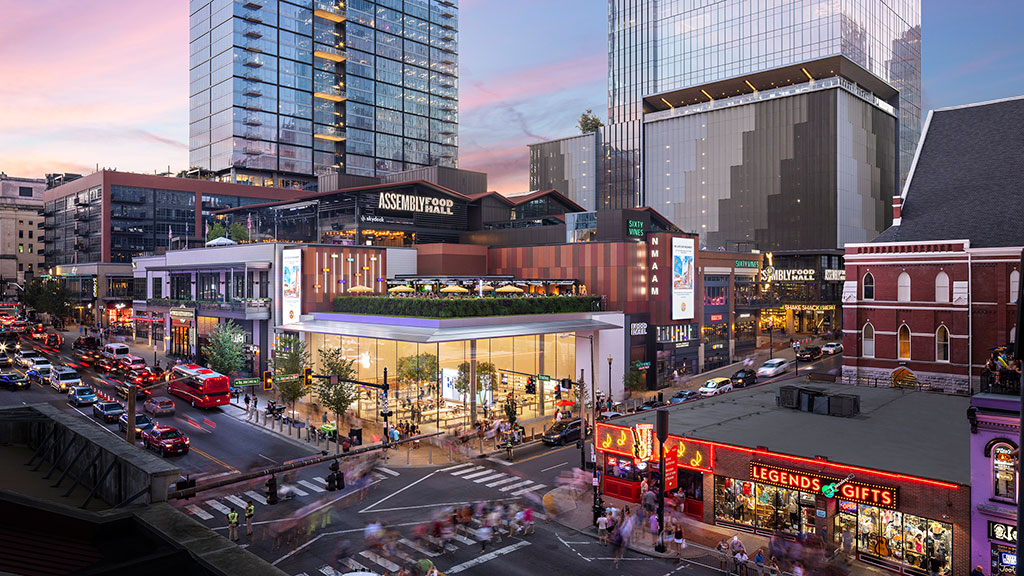This photograph captures the vibrant atmosphere of a bustling city intersection at sunset, transitioning into night. Viewed from a rooftop, the scene is filled with motion as people, dressed in various bright colors, blur into streaks on the crowded streets below. An array of vehicles, including a noticeable bus, trails blurred taillights and headlights, adding to the dynamic energy. Dominating the center is an Apple store, its transparent glass walls revealing a warmly lit interior that glows yellow against the twilight. Surrounding it, a mix of architectural styles is evident—there are older brick buildings and modern glass skyscrapers. The sky, a blend of pink, blue, and gray, casts a magical ambiance over the city. Notable landmarks include a building with a sign reading "Assembly Food Hall" suggesting a lively marketplace atmosphere below, and a vividly illuminated "Legends Gifts" store. The scene is rich with details of urban life, enhanced by the artistic mingling of natural and artificial light.